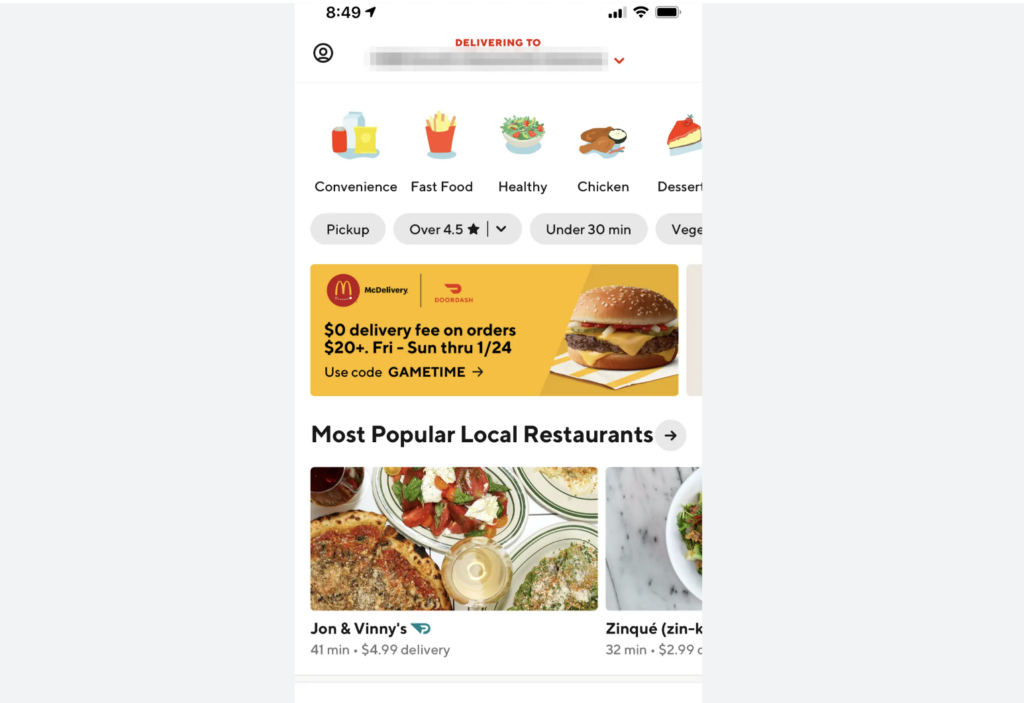The image is a detailed screenshot captured from a mobile phone, presented on a gray background with gray bars on either side. The screenshot itself has a white background. At the very top in black font, the time is shown as 8:49. To the right of the time, an arrow icon indicates location sharing is on, followed by three out of four bars of mobile signal strength, a full Wi-Fi icon, and a fully charged battery icon.

Below the status bar, in red font, the text reads "Delivering to," but the delivery location has been blurred out. The Uber Eats app is open, displaying multiple icons labeled "Convenience," "Fast Food," "Healthy," "Chicken," and "Dessert." Just below these icons, there are several gray ovals with black text reading, from left to right, "Pick Up," "Over 4.5 Stars," "Under 30 Minutes," and "Vegan."

Further down, there's an advertisement for McDonald’s that features a picture of a Big Mac. The ad reads, "McDelivery. Zero delivery fee on orders $20+, Friday through Sunday, 1/24, use code: GAMETIME."

Lastly, at the bottom of the screenshot, in black font, it says "Most Popular Local Restaurants."